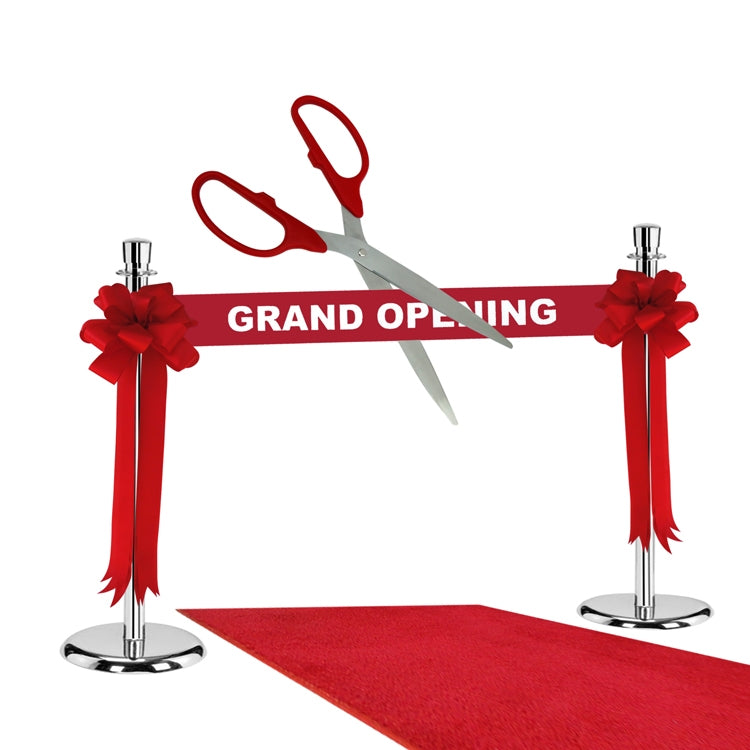The image is a composite collage set against a white background, featuring an exaggeratedly large pair of red-handled scissors poised to cut a bright red ribbon bearing the words "GRAND OPENING" in white, all-capital letters. The ribbon is stretched between two large, silver metal stanchions, adorned with elaborate red rosette decorations and cascading red ribbon. A velvety red carpet lies between the stanchions, leading towards the bottom right-hand corner of the image. The scissors are nearly as tall as the stanchions themselves, which slightly reflect on the ground. The overall scene is a celebratory setup for a grand opening event.